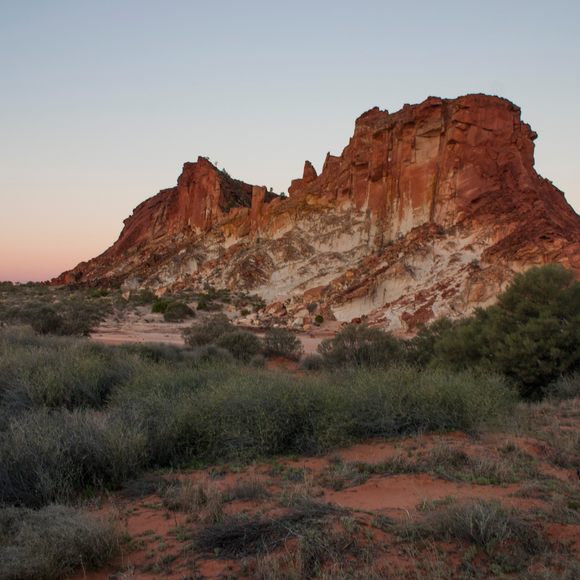The image depicts a rugged, rocky landscape dominated by a large hill or small mountain. The mountain features jagged peaks and is predominantly colored in shades of red, white, and brown, suggesting a clay or sandy composition. It's relatively devoid of trees and appears to be located in an arid or desert-like environment, possibly resembling a scene from the western United States. The surrounding ground is visibly muddy and dirt-covered, interspersed with dark green vegetation and grassy, weedy bushes. The unkempt terrain transitions into sandy ground in the distance. The sky above is light blue, tinged with a pink hue near the horizon, hinting at dusk. There is an overall feel of a remote, untamed landscape that merges both harsh and subtle natural elements.